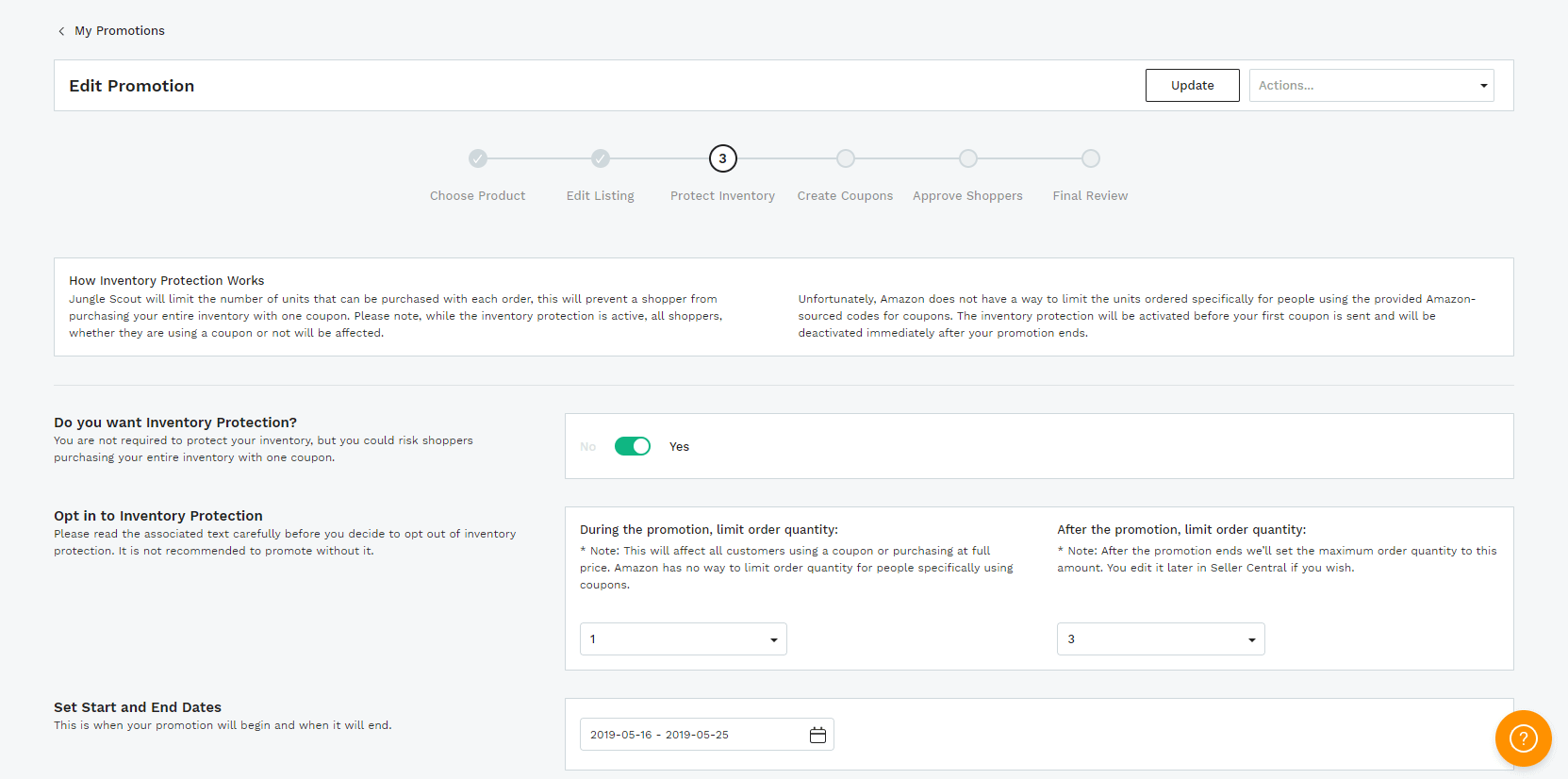This screenshot captures a detailed view of a webpage titled "My Promotions," specifically the "Edit Promotion" section. The image is horizontally oriented, showcasing a series of small black text that is difficult to read due to its size. The page appears to be part of a promotions management tool for a business, offering various options related to inventory and promotional activities.

At the top left corner, the title "My Promotions" is prominently displayed, with "Edit Promotion" directly beneath it. The main section of the screenshot contains several white text boxes with black text inside, providing information about inventory management and protection programs. Users are given the ability to set start and end dates for promotions, indicated by a button featuring date selections.

The navigation steps for setting up a promotion are outlined across the top middle of the page. The steps include "Choose Product," "Edit Listing," "Product Inventory," "Create Coupons," "Approve Shoppers," and "Final Review." Each stage is integral to the promotion setup process.

In the bottom right corner, an orange circular help button with a white question mark is visible, offering user assistance. The background of the page is a light gray color, providing a subtle contrast to the white text boxes.